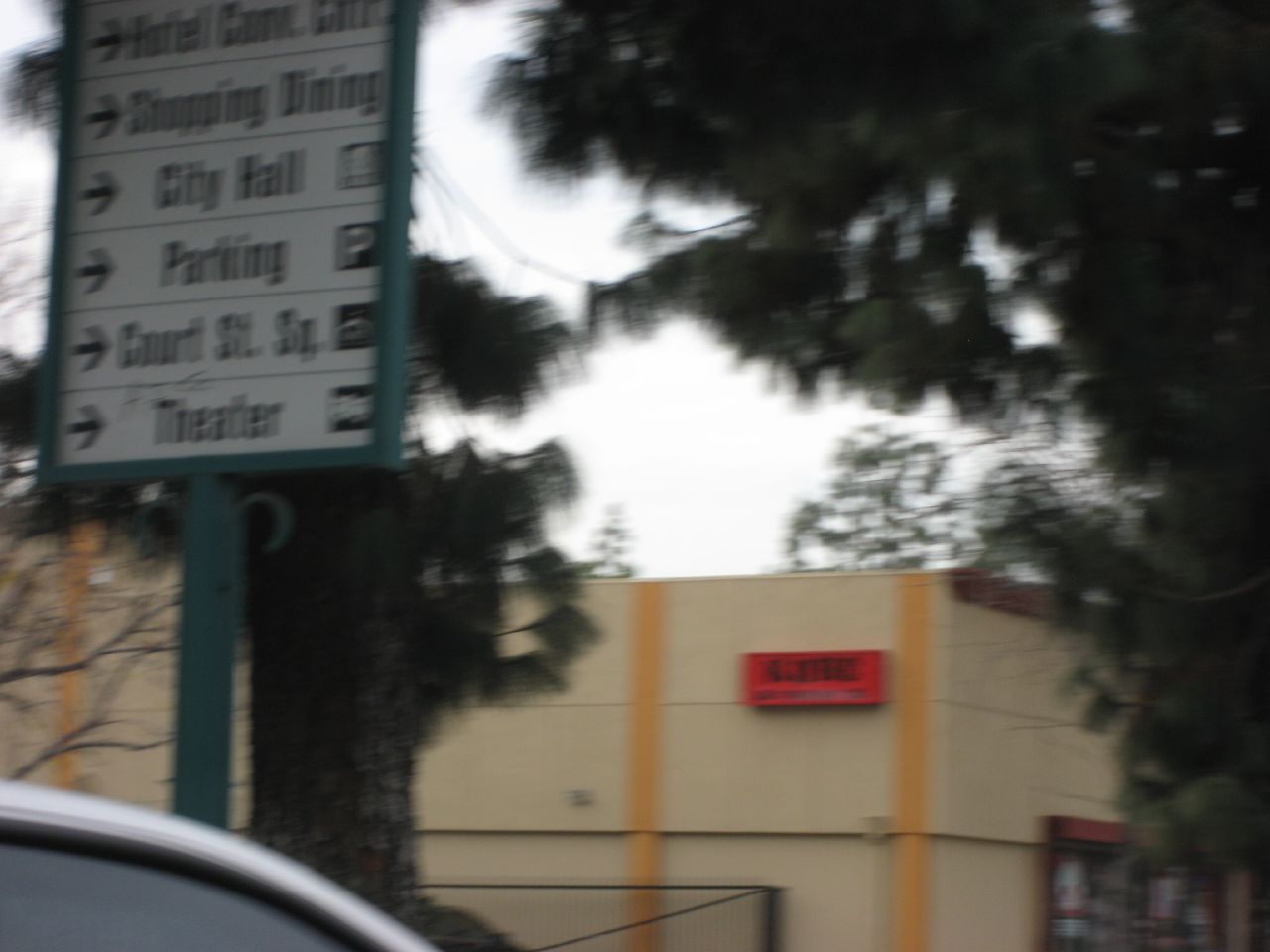In the image, the sky is overcast, casting a white hue across the scene. On the top left, there is a sign that includes directions and icons for "shopping," "dining," and an "airplane," along with references to "my city hall," "court streets," and "my parking." Below this sign, a modest theater is partially visible. The background reveals a building with white walls adorned with vertical yellow stripes. A red rectangle is also noticeable, though its details are obscured due to its angle.

To the right of the building, a large weeping willow tree spreads its branches, adding a touch of lush greenery. The area appears to have well-maintained grass surrounding it. 

In the bottom left of the image, there is a white car parked next to a structure with gray windows. Nearby, an open metal gate can be seen, suggesting an entrance or exit to the depicted area.